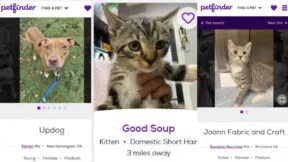This image is sourced from the PetFinder website, which showcases pets up for adoption. The PetFinder logo is displayed in all lowercase cursive letters ("petfinder"). In the left of the image, a beige-colored dog named "Updog" is seen looking up at the camera. Updog is standing in a grassy area, with a blue leash hanging down, connected to an unseen collar.

In the middle, a small kitten named "Good Soup" is featured. The name "Good Soup" is written in purple text, and additional information indicates that the kitten is a domestic short hair and is located three miles away.

On the right side of the image, there is another cat named "Joanne Fabric and Craft." Like the dog, there is a heart icon indicating that someone has favorited Joanne Fabric and Craft, but the kitten in the middle does not have this indicator.